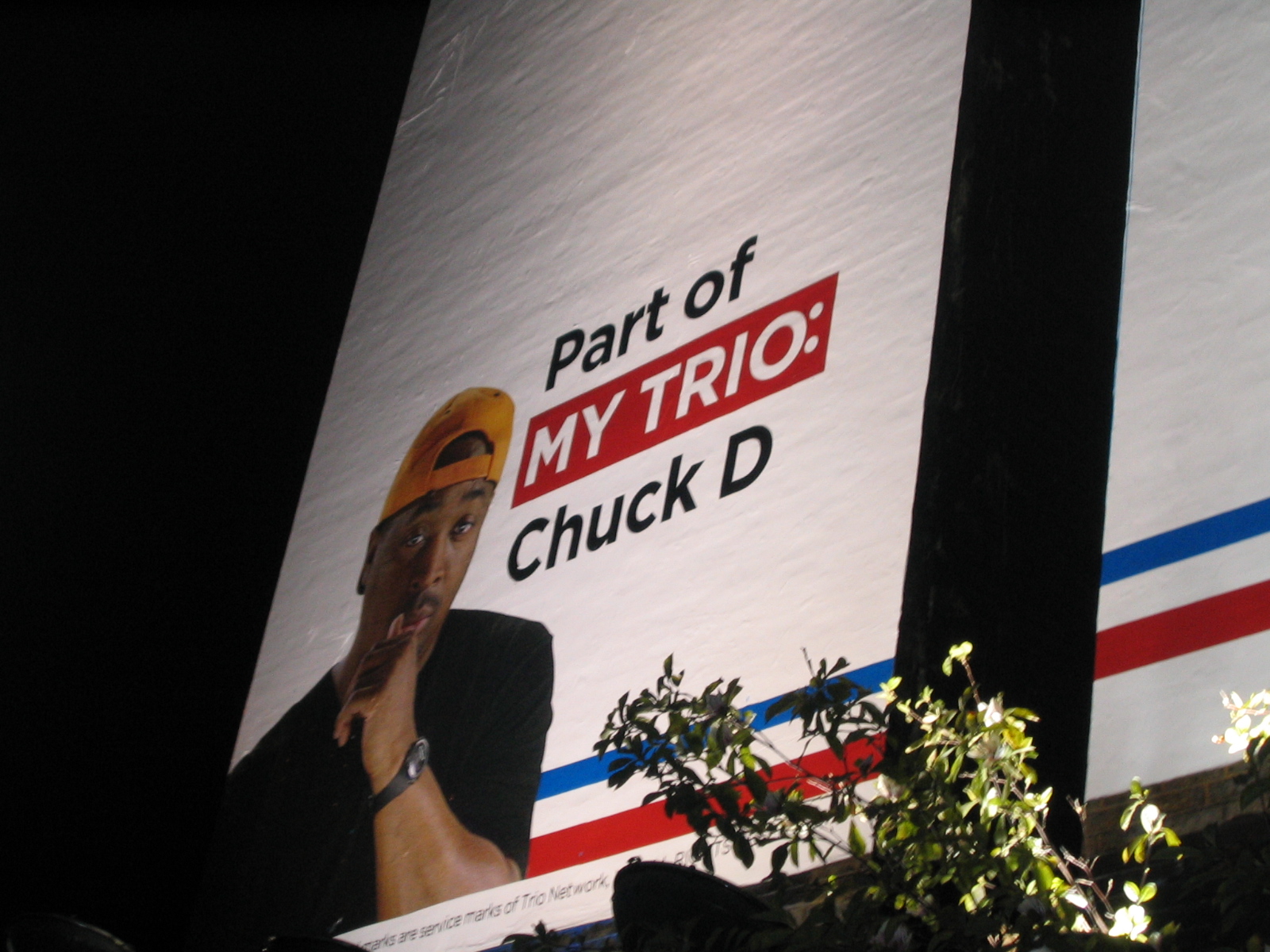The image captures a detailed scene of what appears to be a screencap from a presentation or an outdoor banner. Dominating the image is a large, white banner with the text "Part of My Trio, Chuck D." Overlaid on the banner is a photograph of an African American man positioned on the bottom left. He is wearing a yellow or possibly orange baseball cap backward, a black short-sleeved t-shirt, and a black wristwatch. His left hand is placed by his mouth, and he looks at the camera with raised eyebrows, exuding a thoughtful expression. The background of the banner features a grayish, grainy white texture intersected by horizontal stripes in blue, white, and red, adding a dynamic visual element. Below the text about Chuck D, there’s additional writing partially visible, including the phrase, "Our Service Marks of Trio Network." Adding to the ambiance, outside the screen or banner area, the surrounding space is dark like a theater that has been dimmed, with a thick black vertical bar on the right. A noticeable potted plant with white flowers and lush green foliage sits at the bottom of the frame, lending a touch of nature to the scene.